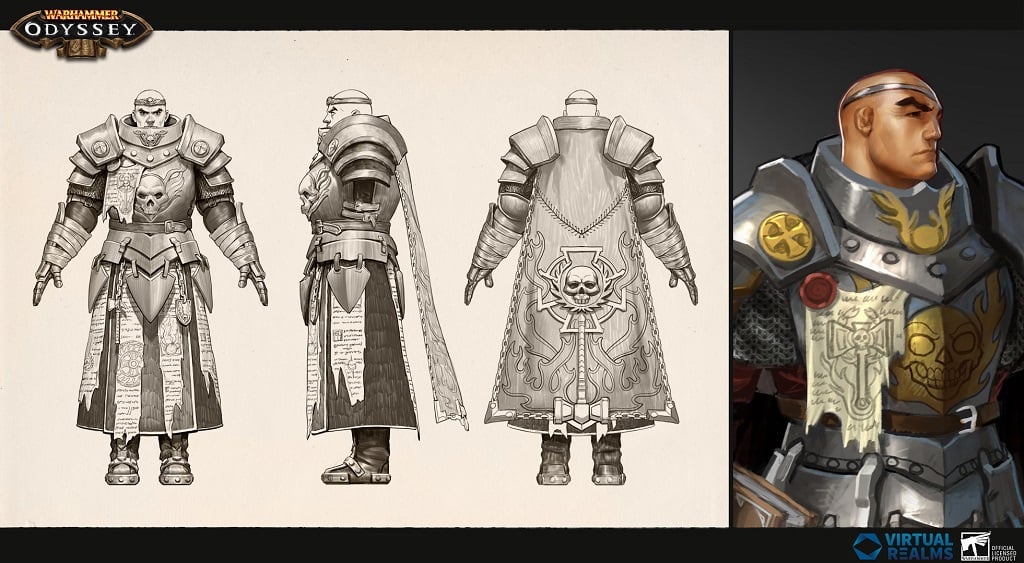This image features character design artwork for the video game Warhammer Odyssey. In the upper left corner, the Warhammer Odyssey logo is prominently displayed, surrounded by a brown border. Below this, the logos for Virtual Realms and Special Licensed Product are visible in smaller fonts. The character depicted is a large, muscular figure adorned in elaborate silver body armor with intricate designs in gold, red, and light brown. A striking detail is the skull chestplate on his armor, complemented by shoulder plates and armor-wrapped wrists. Although the character lacks a helmet, he wears a silver headband. The right side of the image showcases a full-color digital painting of the character's head and torso, emphasizing his robust and protective attire. On the left side, a grayscale character turnaround presents three different views—front, side, and back—highlighting the detailed and multifaceted design of this video game hero.